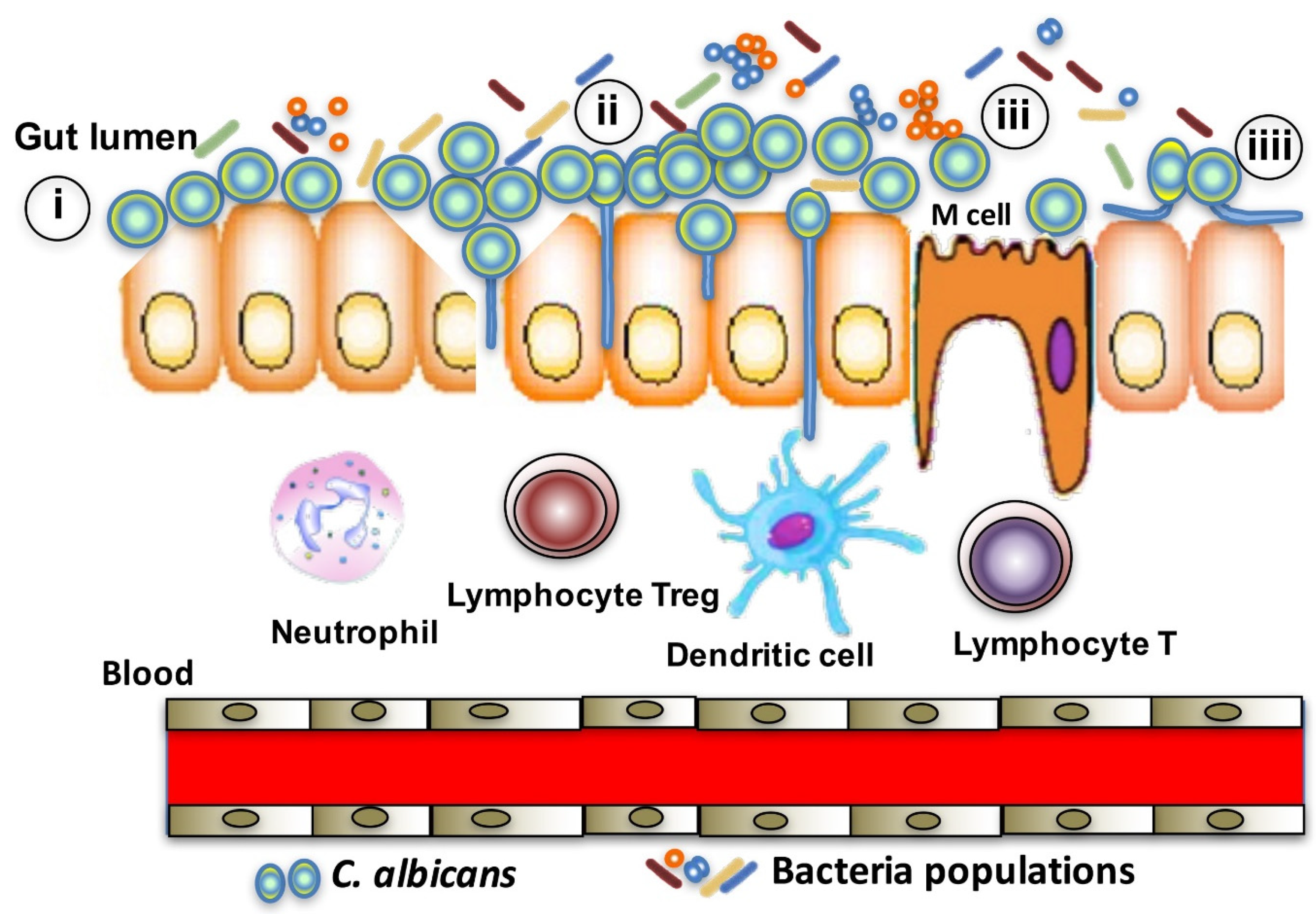This detailed medical diagram, likely sourced from a science textbook, depicts the gut lumen and associated cellular interactions within a human body. The illustration is meticulously color-coded, clearly differentiating various components and cells involved. At the top, the section labeled "gut lumen" showcases a row of structures resembling teeth, interspersed with colorful bubbles and variously shaped figures representing bacterial populations, marked in blue, green, and white. One of these structures, identified as an M cell, sits within a noticeable gap. 

Below the gut lumen, the second segment of the diagram features a horizontal red bar symbolizing a blood vessel, flanked by gray bars, with tan ovals labeled as blood neutrophil, lymphocyte T, lymphocyte Treg, dendritic cell, and bacteria populations. Additional labels include C. albicans, highlighting different types of cells and bacteria commonly observed in the blood. The diagram employs a combination of blue circles, orange rectangles, and other geometric shapes to indicate the presence and interactions of these various cells. The overall style is simple yet informative, most likely computer-animated to ensure clarity and educational value.